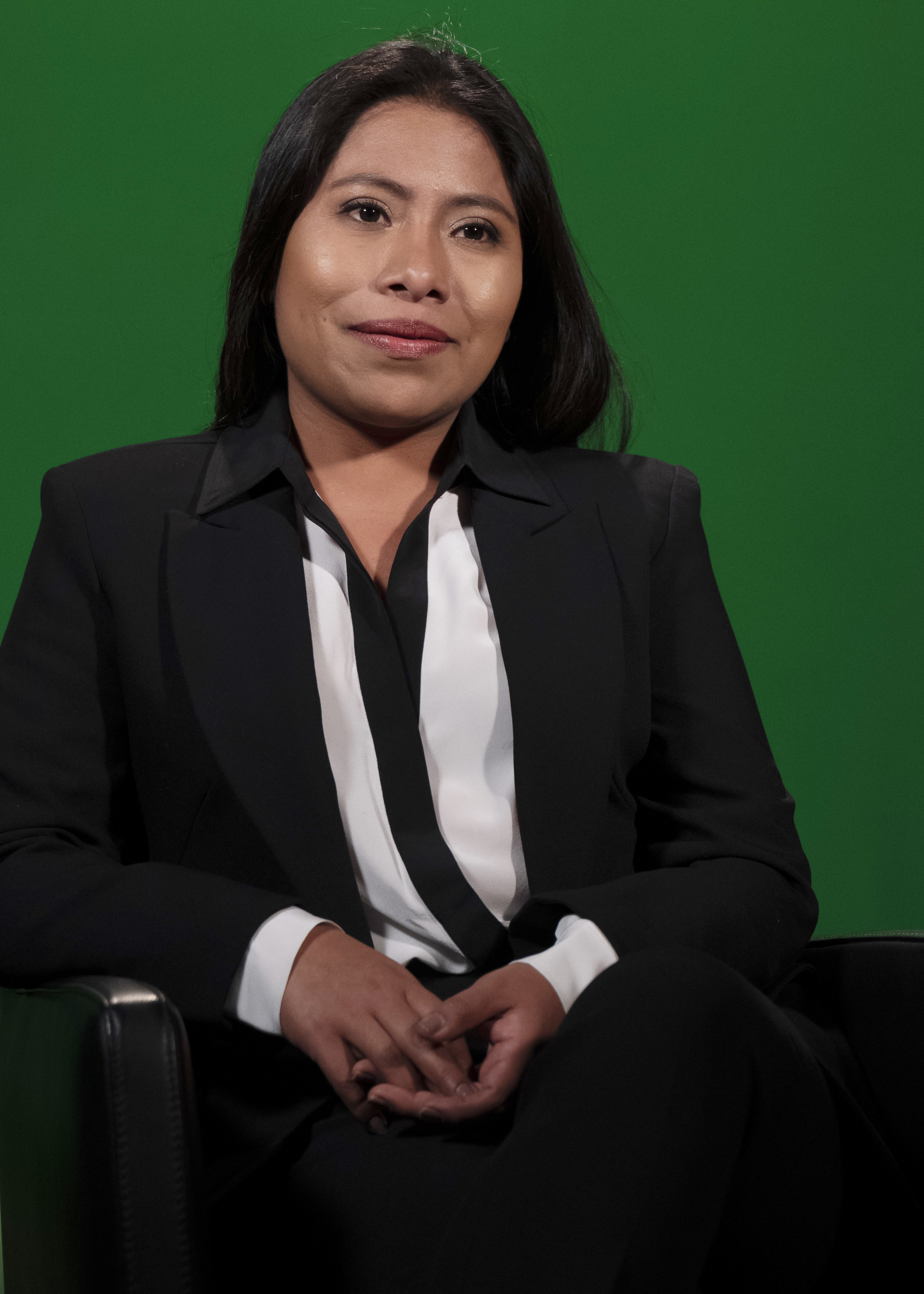The photograph features an Asian woman seated in a low, black leather armchair with thin arms, set against a dark, solid green background. She is dressed in black pants and a black business coat, under which she wears a white blouse with a black collar and a black stripe running down the front closure. The woman has long black hair that extends below her shoulders. She has a serious, almost grimace-like expression and is leaning heavily to one side with her hands interlocked. Her nails are painted a brown color. The image does not show her feet or legs.